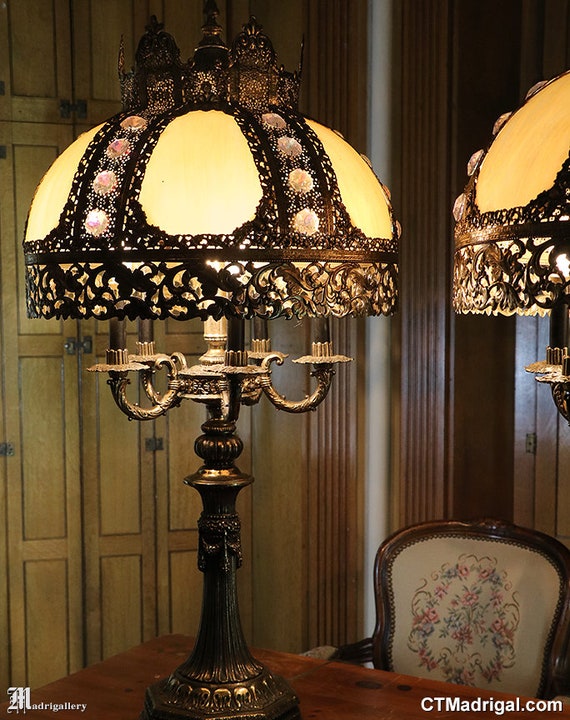This image showcases an intricately designed, antique-style brass table lamp, positioned on a richly finished brown wood table. The lamp features an ornate metal lampshade with a pattern reminiscent of leaves or floral designs, interspersed with frosted glass that emits a warm, yellowish glow. Five bulb sockets, arranged like candle holders, are supported by delicate hooks beneath the shade. In the backdrop, wooden panels and possibly folding doors with a dark brown finish create a refined atmosphere, evoking an old castle or mansion. A chair with a dark brown wooden frame and white cushioned upholstery, decorated with floral embroideries in pink and blue, is positioned near the table. In the corners of the image, the text “Madrigallery” and the website address “ctmadrigal.com” are visible, adding to the elegant, vintage ambiance of the setting.